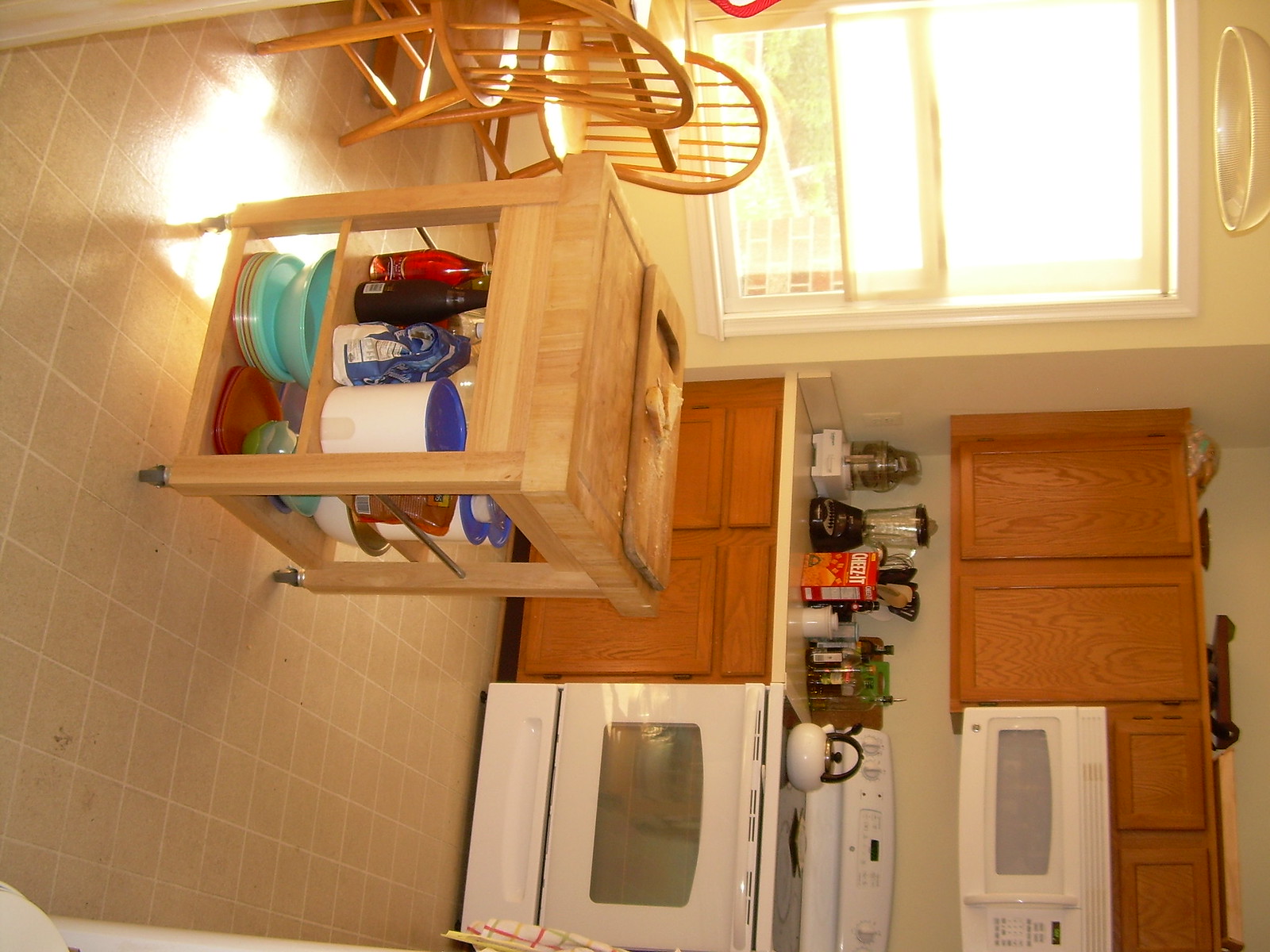In this brightly lit kitchen scene, sunlight pours through a window, illuminating the space in a warm, daytime glow. The kitchen, rotated on its side in the photograph, features light-colored walls and is furnished with oak cabinets both above and below the countertops. The white appliances include an electric stove with a ceramic cooktop and a microwave. On the stove sits a tea kettle, while the light-colored countertops are adorned with various items such as a blender, kitchen utensils, and a box of Cheez-Its. 

A mobile butcher block island, made of oak and complete with a cutting board on top, stands prominently in the room. This island features two shelves stocked with typical kitchen supplies, including bottles and bowls. Partially visible in the frame, an oak table and a couple of chairs hint at a cozy dining area. Overall, the detailed arrangement and the abundance of natural light contribute to a warm and inviting kitchen atmosphere.